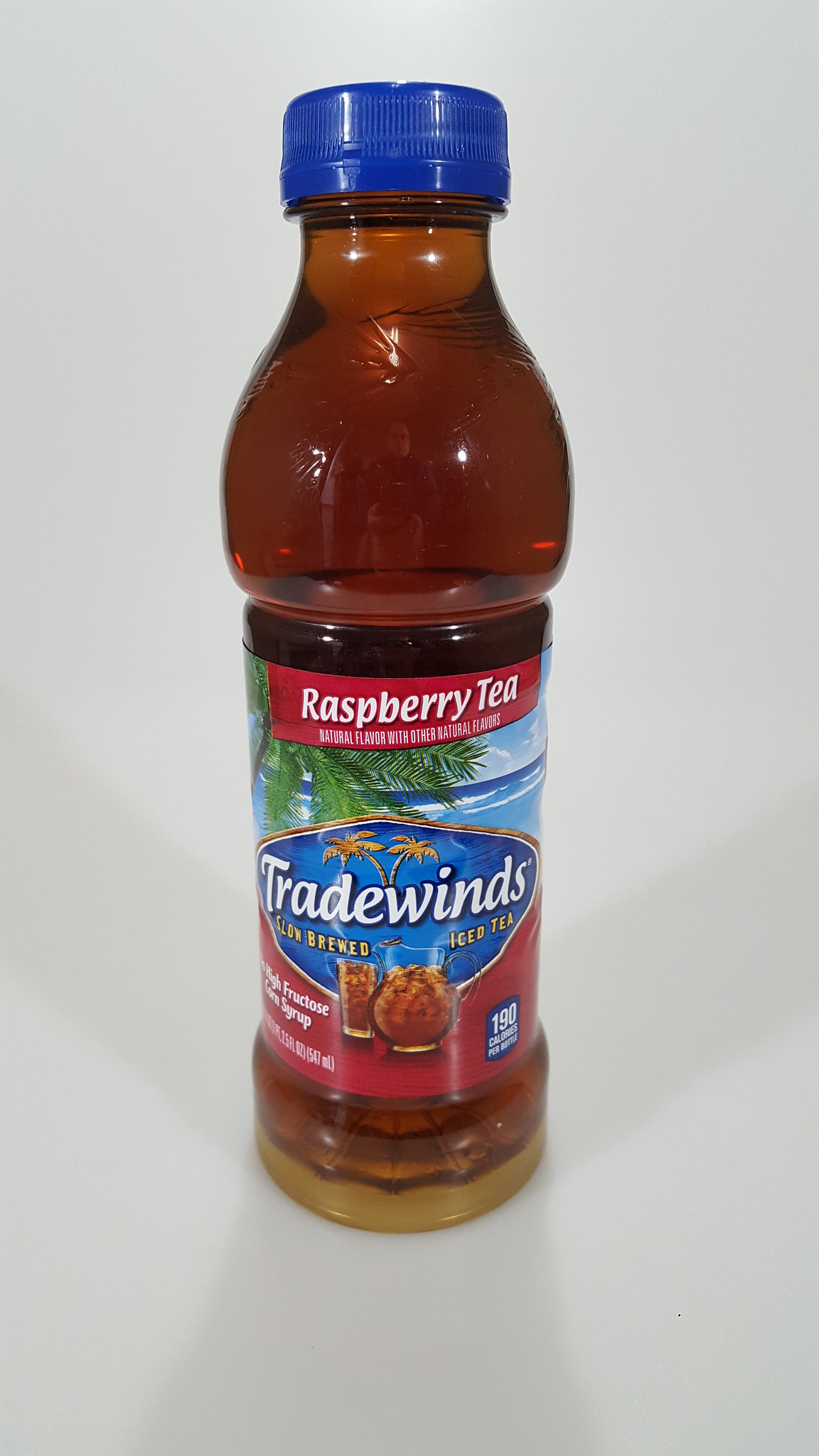This image features a single plastic bottle with a clear body, capped by a blue screw-on lid, and filled with a brownish liquid. The bottle is set against a white background, casting natural shadows, indicating it was photographed in a professional setting. The label wrapped around the bottle is vibrant and detailed, predominantly featuring red, blue, and green hues. At the top of the label, a burgundy-red banner displays the words "Raspberry Tea" in white letters, followed by "Natural Flavors with Other Natural Flavors." Prominently on the label is the "Tradewinds" logo, which includes white text set against a blue backdrop, highlighted by two palm trees. The background of the label showcases a picturesque scene with blue water, blue skies, and white clouds, enhancing the tropical theme. Also depicted on the label is a glass and a pitcher of iced tea filled with ice, symbolizing the beverage inside. At the very bottom of the label, the calorie content is indicated as "190 calories." The overall aesthetic suggests that this image aims to present the product attractively, possibly for use on a website or in marketing materials.